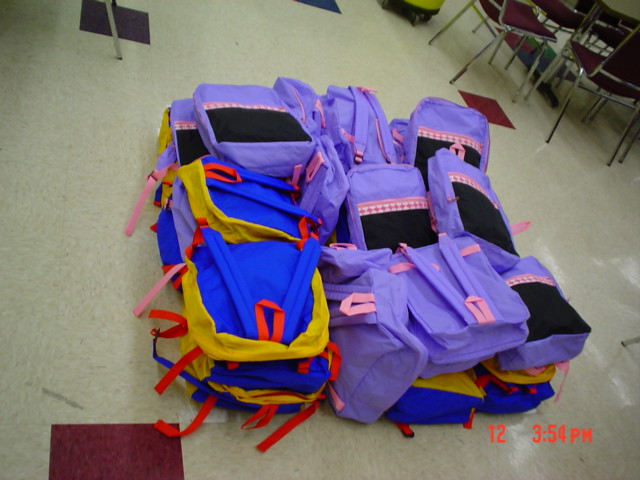This is a photograph taken indoors, possibly in a school cafeteria or classroom, under poor artificial lighting, with a cream white floor featuring random maroon, red, and brown squares scattered throughout. In the image, there is a neatly organized pile of new backpacks, forming a roughly square shape. The floor surrounding the pile shows noticeable scuff marks, including a distinct black scratch in the lower left corner. In the upper right corner, red chairs and a table are partially visible, while the upper left corner shows the leg of a chair. 

The backpacks in the foreground are primarily two types: the first type is blue with yellow sides, orange straps, and a red loop likely for hanging. The second type is light purple with pink edges, a black front panel accented by a pink and white checkered strip, and pink buckles on the straps. Additionally, there’s a superimposed text displaying the number "12" and the time "3.54pm" in red located in the lower right corner of the image.